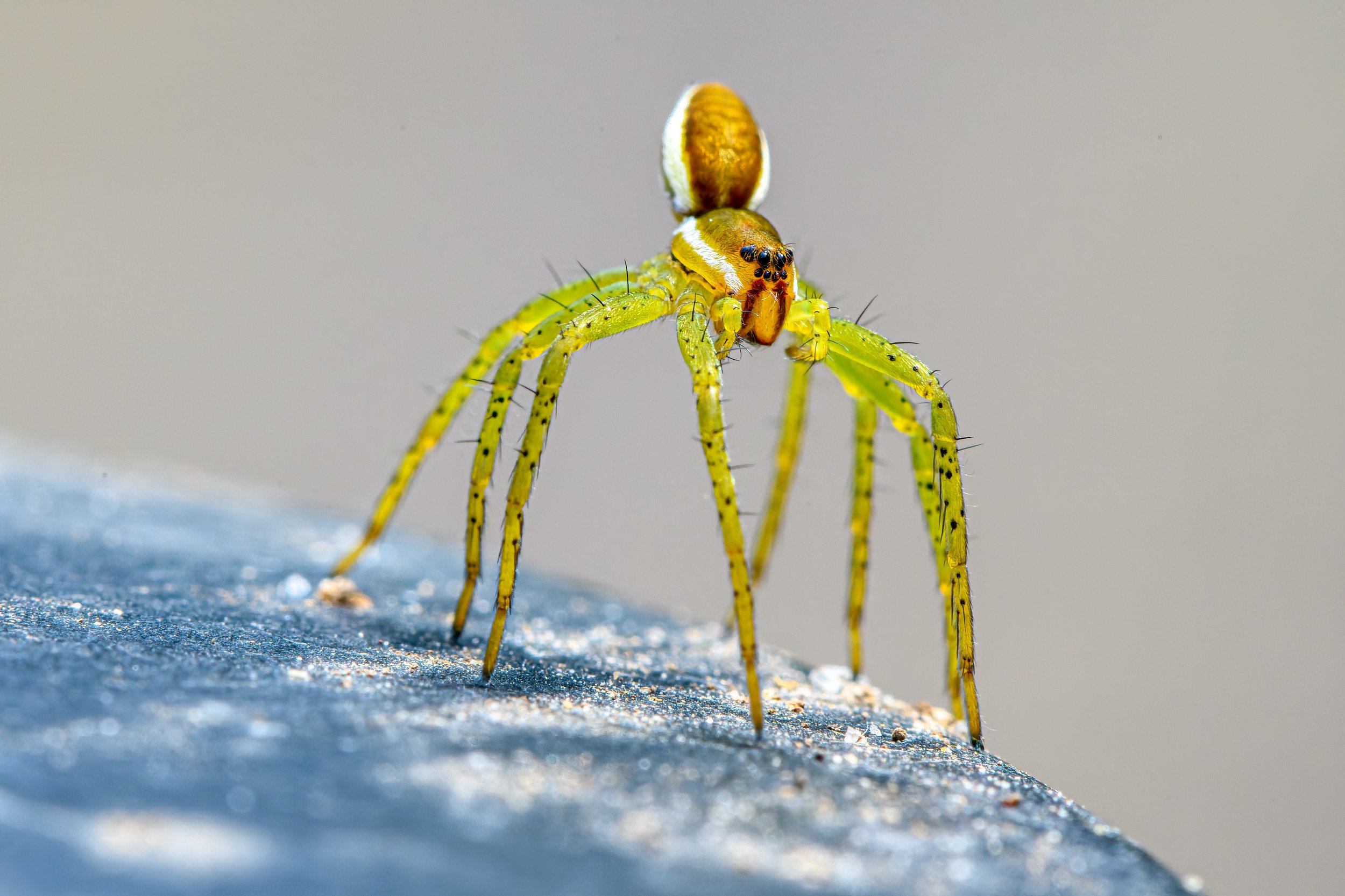This is an extreme close-up photograph of a spider with strikingly long, thin, neon yellowish-green legs that appear almost transparent. Each leg has small black spiky hairs and black dots, and they shimmer with hints of gold when viewed from certain angles. The spider's body features a dark golden brown hue with distinct white stripes running along each side and across the face. The focused image captures its multiple black eyes, giving it a somewhat intense expression. There are tiny red lines near the mouth area. The spider is perched on a bluish-gray, shiny surface that resembles a round rock or crystal, with bits of dust or dirt scattered on it. The background of the photograph is blurry and gray, emphasizing the vivid details of the spider and its peculiar, rocky platform.